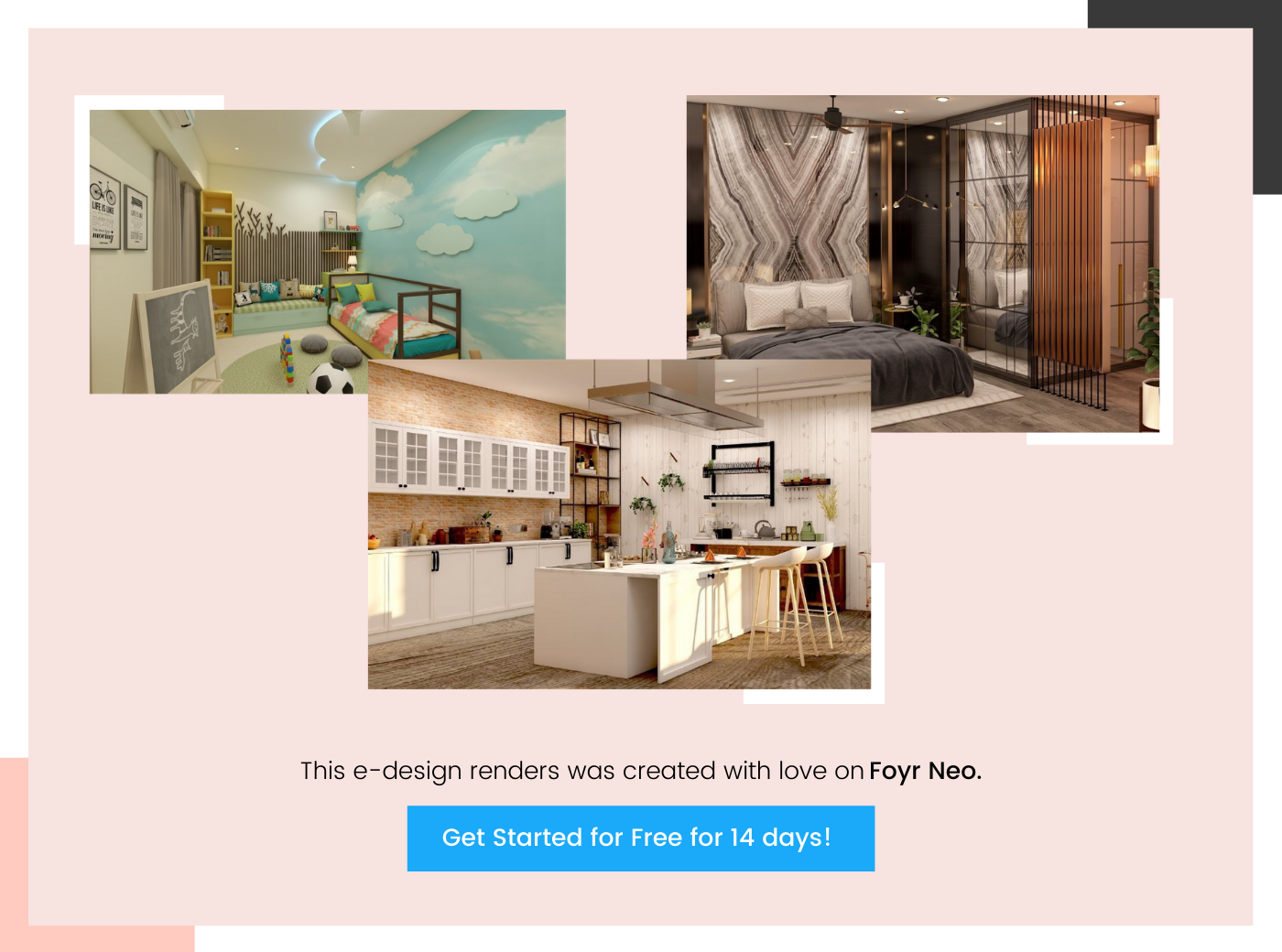The image depicts a promotional banner from the website Foyer Neo. The background is a soft light pink, featuring two highlighted areas: the top right corner in black and a tiny highlight in the lower left corner in pink. Within these highlights, three overlapping images are displayed, each showcasing different interior design renderings created with the Foyer Neo platform.

The first image presents a well-decorated children's room. It includes a small bed, a cozy carpet, a blackboard, and a blue wall adorned with playful cloud drawings. Ample storage space and various decorative items are also visible in the background.

The second image highlights a modern kitchen area. This scene features a polished kitchen counter with seating arrangements, sleek cabinets, a spice rack, and elegant wooden flooring, showcasing both functionality and style.

The third image showcases a luxurious master bedroom. Key elements include a partial view of the closet area, a see-through glass door, and a bed dressed with a grey duvet. The backdrop behind the bed has a marble-like texture, adding a touch of sophistication.

Below these images, a text reads: "This eDesign render was created with love on Foyer Neo," with "Foyer Neo" emphasized in bold. A blue button beneath the text invites users to "Get Started for Free for 14 Days," suggesting an easy signup process for a free trial on the website.